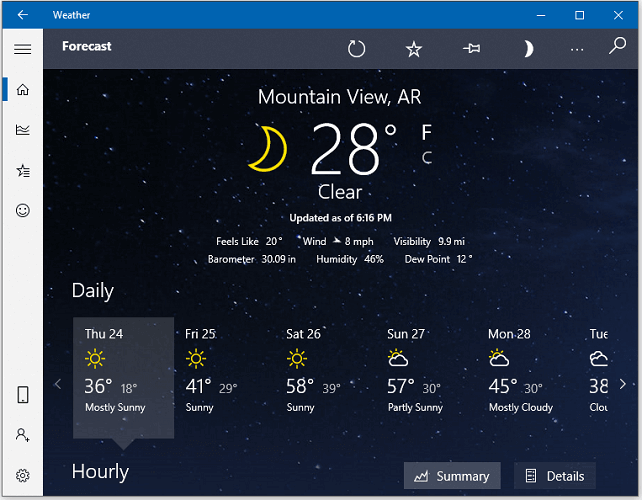This screenshot, seemingly from a weather website, exhibits a detailed layout highlighting both the navigation and weather information. At the very top, a blue bar features a back button on the left, with "Weather" written in the center, and buttons for minimizing, maximizing, and closing the window on the right. Directly below is a concise black bar with buttons labeled "Forecast," "Refresh," "Star," "Pin," "Moon," and icons for additional options as well as a magnifying glass for search functionality. 

A white side menu on the left includes various icons such as a house (home), water drop, star, smiley face, flag, person, and settings, with the home icon currently highlighted by a blue slider.

Center stage on a dark, starry background, the screen prominently displays the weather details for Mountain View, Arizona. Here, an icon of the moon is shown along with the current temperature of 28 degrees Fahrenheit and a clear sky description. Below, a brief forecast spans from Thursday through half of Tuesday, followed by an 'Hourly' section for more specific updates.